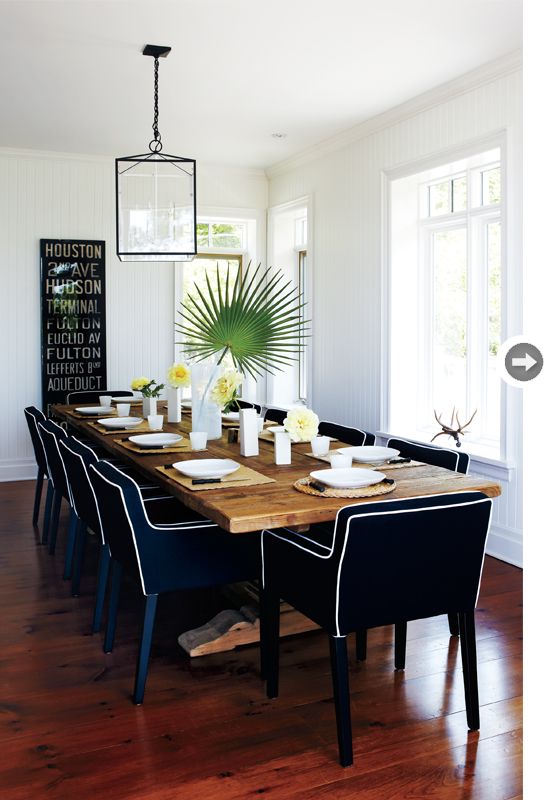The photograph depicts a modern dining room with a sleek, contemporary design. Dominating the center of this vertical rectangular image is a long wooden table with metal legs, complemented by black leather chairs, which feature white trim and metal legs. The table is adorned with pristine white plates and cutlery, set atop a carpet. A large, lush palm plant, distinguished by its numerous needle-like leaves, sits in the middle of the table, flanked by four white vases containing yellow flowers. Overhead, a cubic light fixture with visible bulbs hangs from the ceiling, illuminating the space.

The room is bathed in natural light streaming through multiple windows with drawn curtains, emphasizing the brightness outside. The walls and ceiling are pure white, contrasting with the dark, richly-colored wooden floor. On the far left wall, a black frame with visible text fragments such as "Houston Avenue," "Hudson Terminal," and "Fulton Letters" adds an artistic element. The overall ambiance exudes cleanliness and modern elegance, accentuated by the clear chandelier and the reflective light on the wooden floors.